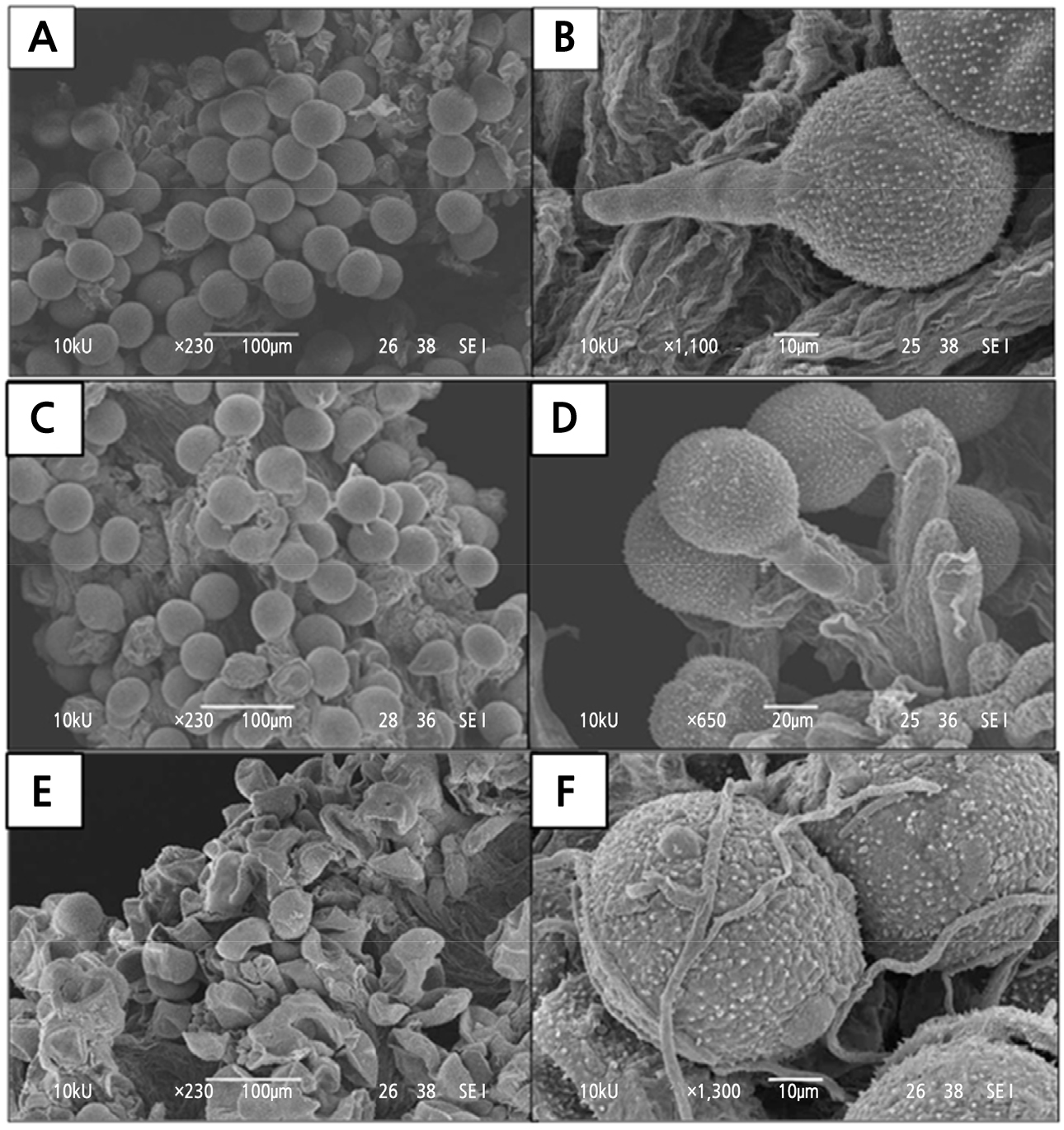The image is a detailed black and white depiction of six microscopic photographs arranged in three rows and two columns, labeled A through F. Each label corresponds to various cell clusters and individual cells observed under a microscope. The cells appear as round, gray circles against a dark background.

- **A** shows a cluster of round cells with a lighter edge around each cell and detailed measurements including "10Ku," "230x," and "100 micrometers."
- **B** presents a close-up view of a single cell with a distinctive tail, and similar measurements like "10Ku," "1100x," and "10 micrometers."
- **C** displays more of the same cells as in A but in a brighter shade.
- **D** features an enlarged view of a cluster of the round cells with tails, similar to those in B.
- **E** depicts a section of deflated, damaged cells.
- **F** shows cells with additional wiggly lines covering them. 

Across all images, the texture and structure's details are visible, emphasizing microscopic clarity and precision. The dimensions and magnification levels are marked on each photograph, suggesting careful documentation and scientific analysis.